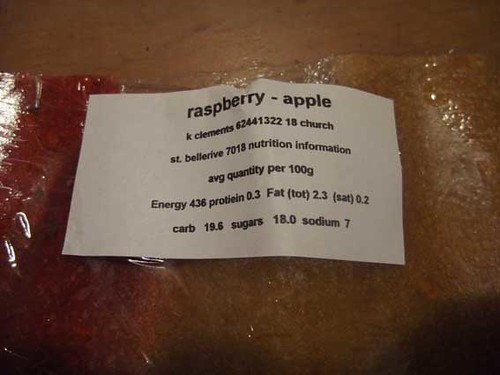A square-shaped image features a white paper centered against an unspecified background. The paper displays black text, presenting information in a structured format. At the top of the paper, it reads "Raspberry-Apple" in bold letters, indicating the flavor or main ingredient. Beneath this, the text includes the name "K. Clemens" alongside numerical sequences: "6244 1322," followed by "space 18 church." Further down, a line specifies "st.embellireve 7018," which could refer to an address or a brand name. The document also includes nutrition information, listed as "avg quantity per 100g," and provides specifics such as "energy 436," "protein 0.3," and "fat (tot) 2.3," where "tot" is enclosed in parentheses.